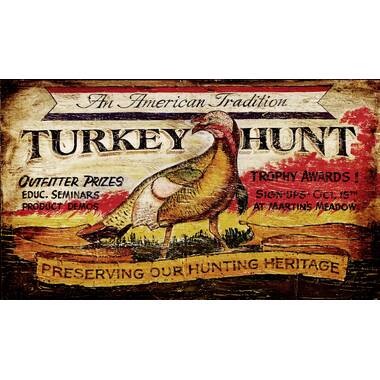This detailed advertisement illustration, seemingly hand-drawn and painted with a vintage touch, promotes an event titled "An American Tradition: TURKEY HUNT" in large, capital letters. The focal point of the image is a centrally positioned turkey, depicted with meticulous detail. The bird has tight, multi-colored feathers and a prominent red wattle hanging under its beak. It stands in a grassy or wheat field, facing right but glancing left. The artwork employs a palette of earthy tones including beige, brown, gold, and red, alongside hints of a possibly red sunset in the background.

On the left-hand side, the text outlines various highlights of the event: "Outfitter Prizes," "Educational Seminars," and "Product Demos." On the right-hand side, it mentions "Trophy Awards!" and provides event sign-up details: "Signups October 15th at Martin Meadows." At the bottom of the illustration, an emblem reads "Preserving Our Hunting Heritage," reinforcing the theme of cultural tradition. This rich, antique-style illustration encapsulates the essence of American hunting heritage and invites participants to engage in the event.